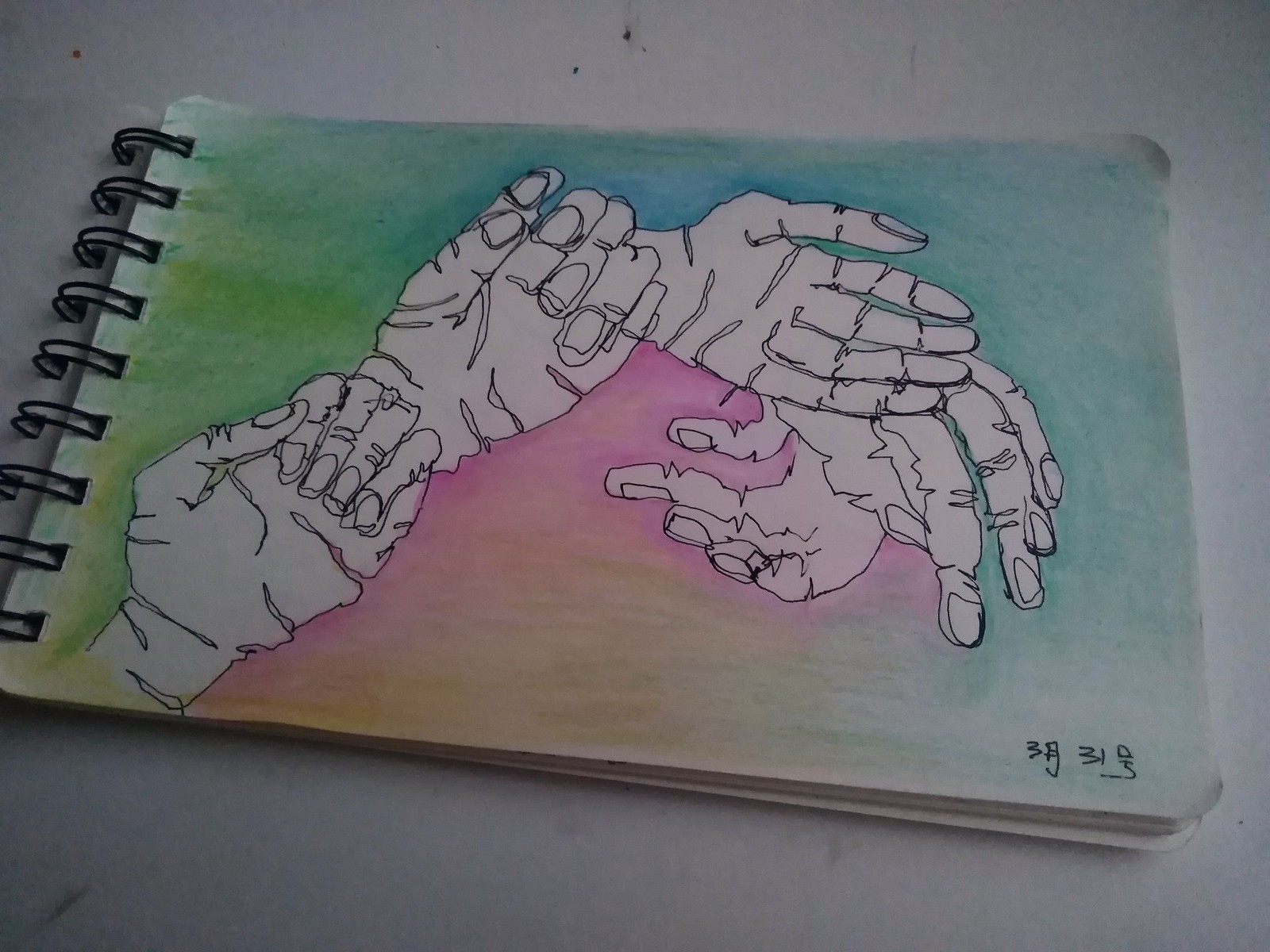The image showcases a meticulously hand-drawn and colored artwork set on a paper pad, distinguished by its eight black double spirals binding along the left side. The pad occupies most of the frame and rests atop a pristine white table. The artwork itself features a vibrant blend of colors, with green hues primarily on the left side transitioning into a dominant blue that envelopes the top and right sections of the drawing. Emerging from the bottom of the piece are five detailed hands, each with fingers outstretched and interconnected in an arching formation, reminiscent of a rainbow. These hands start from the bottom left, ascend towards the top, and curve back down towards the bottom right, with one hand prominently curving inward and pointing four fingers towards the center. The hand nestled just beneath the shaded area boasts a striking color gradient, transitioning from pink to orange, adding a rich, dynamic contrast to the overall composition.